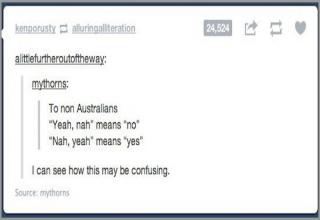In the image, a small screenshot is displayed showing a snippet of a Tumblr post. At the top left, the username "KENPORUSTY" is visible, indicating the individual who has reblogged the post. The original post appears to be from another user, though their username is obscured and difficult to decipher. The post has been reblogged 24,524 times, as noted next to sharing icons for reblogging, liking, and other sharing options.

Below this line containing the post's metrics, additional usernames are displayed, both underlined. One username, "A Little Feather Out of the Way," is written in black text. Following this is another underlined username, "My Thorns." The text they are reblogging reads: "For non-Australians, 'yeah nah' means no. 'Nah yeah' means yes." Beneath this, a reply is added which states: "I can see how this may be confusing."

The layout captures the essence of Tumblr's interactive features, showcasing the user engagement and the layered conversational nature of reblogging and replies within the platform.